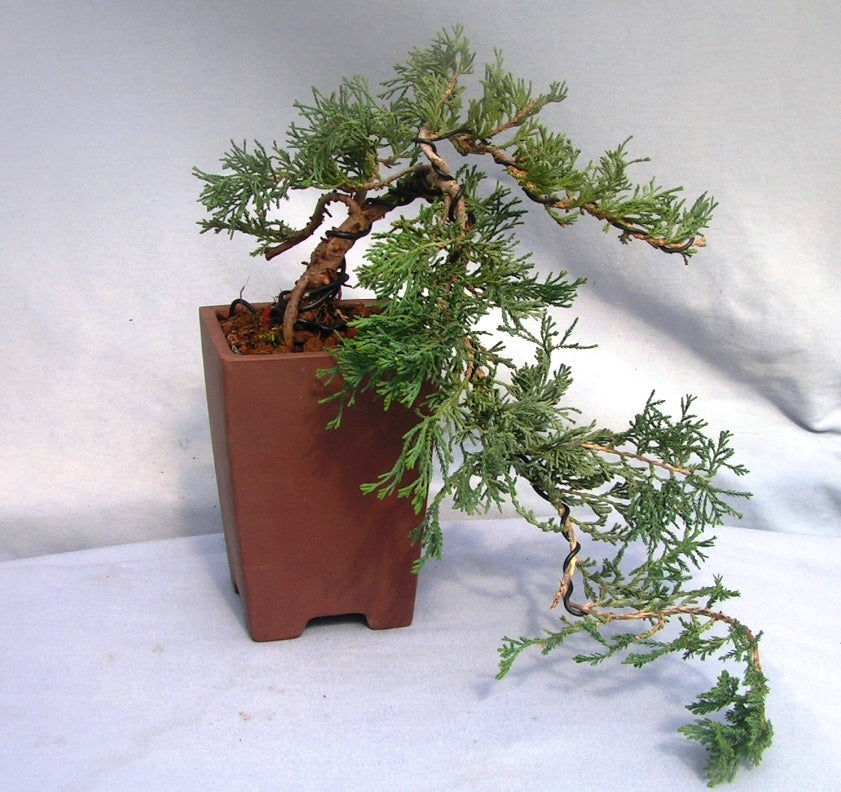In this square-shaped color photograph, a bonsai tree is prominently featured, set against a white, slightly wrinkled fabric background, reminiscent of a studio setting. The bonsai, resembling a cedar tree, is housed in a tall, rectangular brown pot, possibly terracotta, about eight inches high. The tree itself has a gnarled, ancient-looking trunk that twists and bends downward, seemingly supported by a piece of wire to achieve its trailing shape. The greenery comprises thick, needle-like leaves that extend outward and hang down, almost touching the white fabric-covered surface beneath. The overall presentation emphasizes the intricate, delicate nature of the bonsai, with attention to its rustic charm and unique form.